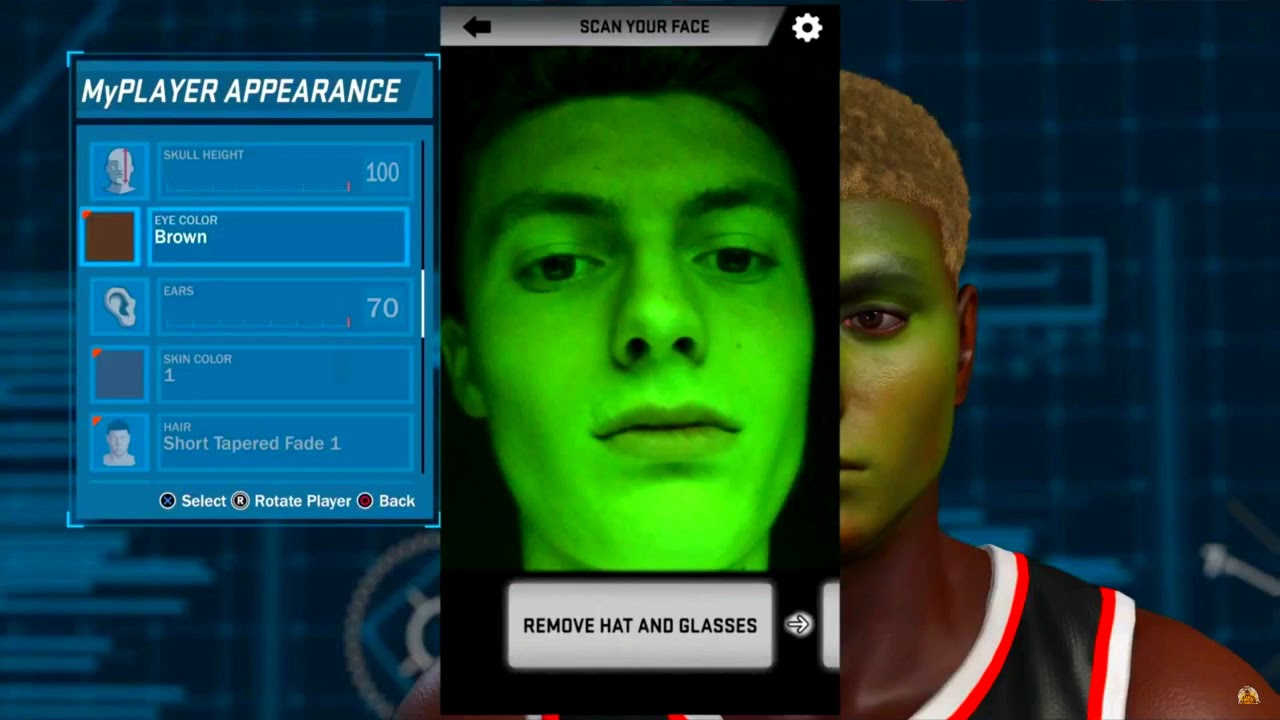The image showcases the avatar creation pop-up for a video game, set against an indigo background typical of gaming interfaces, adorned with vaguely science-fiction symbols and icons. The partially visible cartoon-style avatar has brown skin and is donning a black jersey with red and white borders. Notably, the avatar has an afro-style hair that glows in a comic book graphic style and bears a bronze hat. The avatar’s left eye to the start of the nose is visible, while the rest is obscured by a pop-up window.

The pop-up is titled "Scan Your Face," and features a neon green, slightly angled human-like face icon beneath the heading. Instructions in the pop-up advise players to "Remove hat and glasses." A gear setting icon is located in the top right corner of the pop-up.

Adjacent to this is another pop-up titled "My Player Appearance," offering customization options. These options include:
1. Skull height, set at 100.
2. Eye color, displayed as brown.
3. Ears, represented by a graphic image of an ear with a notation of 70.
4. Skin color, shown as a dark red square with a small red dot, labeled with the number 1.
5. Hair, listed as "short tempered fade 1," accompanied by an icon showing a head and shoulders with a red dot at the top.

Upon loading these settings, selecting "Rotate Player" allows users to see the modifications.